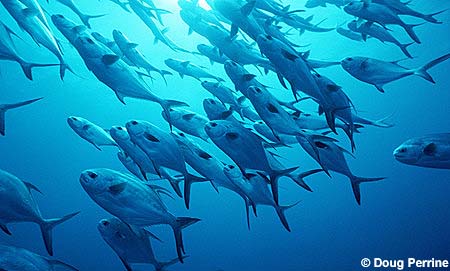This underwater photograph, credited to Doug Perrine, captures a mesmerizing scene of a school of around 50-60 fish swimming in unison in a vibrant, clear blue body of water. The fish, varying in size with both adult and juvenile members, exhibit a light body with darker, likely black-tinted fins. They are closely clustered, all moving in the same upward trajectory towards the left, as sunlight streams down from above, illuminating the depths and adding a glistening effect to the scene. The fish, resembling smaller versions of sunfish with their large, oval-shaped, flat bodies, present a tranquil yet dynamic movement as they navigate through the underwater world.